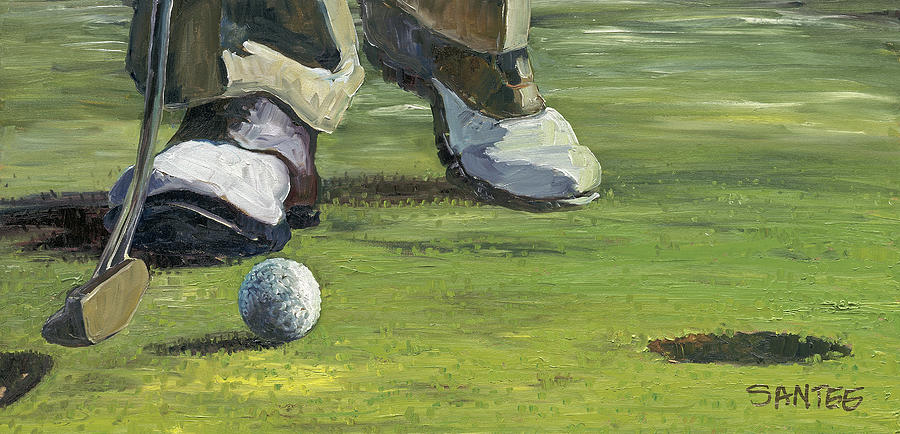This freehand-painted image captures a golfer in the midst of a putt on a verdant golf course. The scene is viewed from a low angle, emphasizing the golfer's brown and white saddle shoes and the tan khaki pants visible at his ankles. The golfer's putter, silver with a brownish head, is poised near a white ball rolling towards a conspicuously large hole approximately eight inches away. The golf course's green hues are meticulously shaded, with horizontal line work adding an impressionistic texture to the grass and dirt. The backdrop remains minimalistic, offering no sight of other golfers, thus focusing entirely on the singular action. The painting is signed "Santee" in brown paint on the lower right-hand corner, adding a personal touch to the artwork. The precise detailing of the scene—down to the distinct footwear and the calculated shot in progress—provides a vivid, lifelike representation of a tranquil moment in the sport.